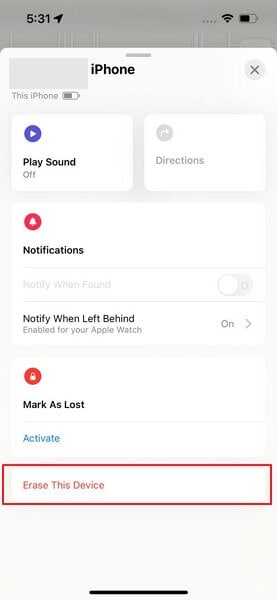This image is a screenshot from an iPhone, displaying a feature for managing the device's settings remotely. At the top, the interface is identified with the label "iPhone" in bold black letters on a gray strip. The status bar at the top shows the current time (5:31), battery life, and connection status, indicating a strong signal. 

Below this, there are several control options. The first section offers a "Play Sound" feature, which is currently toggled off. The next section provides "Directions." Underneath that, there's a "Notifications" section marked with a red circle, which indicates that notifications are enabled for the Apple Watch. This section states "Notify When Left Behind" and is set to "On."

Further down, there's an option labeled "Mark as Lost," accompanied by a blue "Activate" button, allowing the owner to mark the device as lost if necessary. Lastly, at the bottom is a prominent red box with white text that reads "Erase This Device," offering the option to remotely erase all data on the iPhone for security purposes.